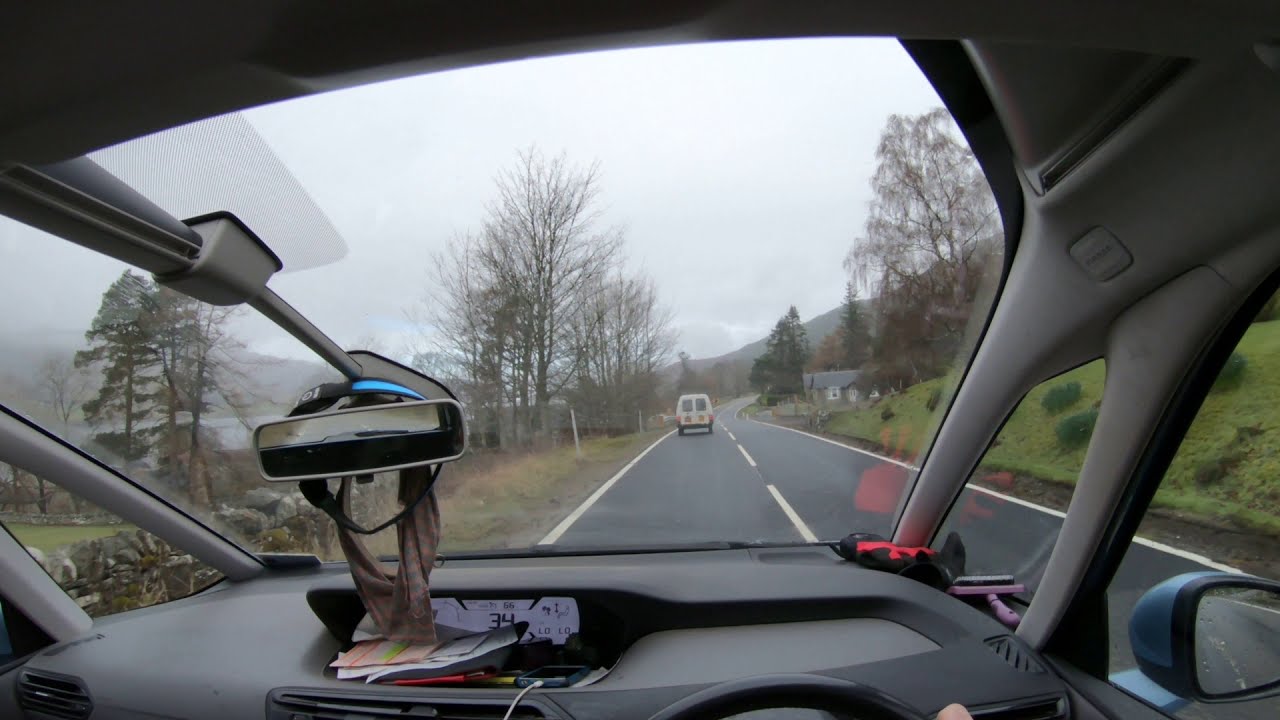The photo captures an interior view from inside a grayish car, featuring a cluttered dashboard with various items including a cell phone with a charger, scattered papers, and a red object. Hanging from the central rearview mirror—possibly draped with a cloth—are additional items. A glove rests on the right side of the windshield. The image is taken through the front window on a narrow, winding road marked by broken white lines, with a white van visible ahead. On the left side of the road, you can see descending terrain with dead grass, a fence, and leafless trees, indicating late fall or winter. The right side of the road features ascending green hills with darker green bushes. The background reveals an overcast sky, adding to the hazy atmosphere. Further ahead, a house with a dark roof is visible, with distant mountains silhouetted against the cloudy, white sky. This scene possibly suggests a drive through a European countryside judging by the left-hand driving orientation.